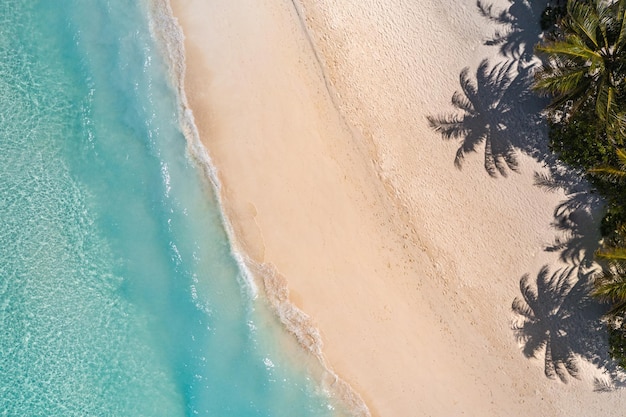This aerial image captures a serene, white sandy beach meeting crystal-clear, aqua green ocean waters. The left side of the photograph showcases calm, foamy waves rippling gently towards the shore. The sand, light in color and smooth towards the water's edge, transitions to a typical sandy texture further inland. On the right side of the image, a cluster of plush, dark green palm trees cast distinct shadows onto the beach. The overall scene, bathed in sunlight, features the trees' shadows vividly etched into the sand, adding to the tranquil and picturesque coastal landscape.